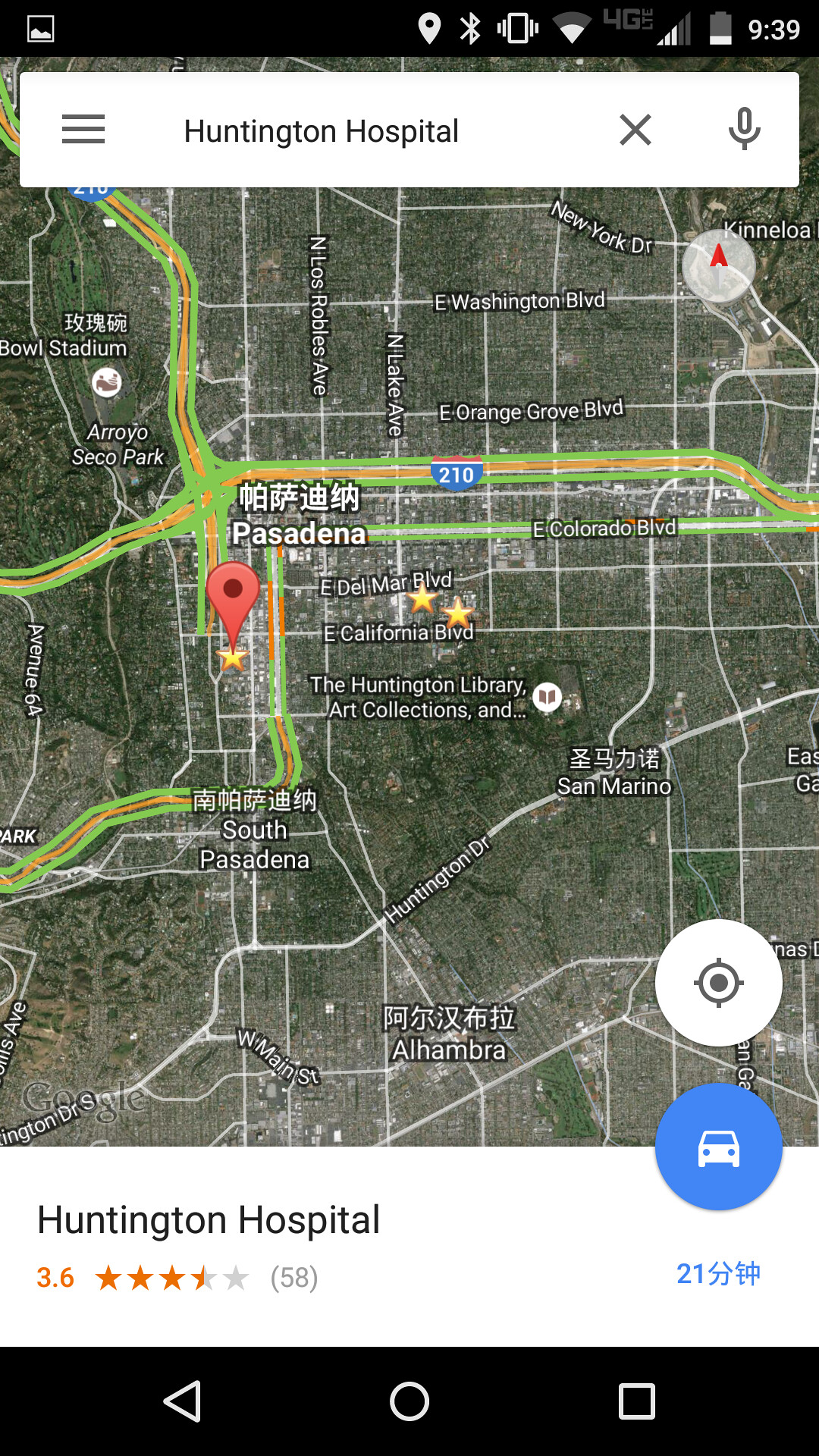This screenshot captures a detailed bird's eye view of Huntington Hospital on Google Maps. The hospital is centrally located within the image, surrounded by neighboring areas. In the bottom left corner, "Huntington Hospital" is labeled, accompanied by an orange rating of 3.6 stars based on 58 reviews in grey text. To the right, the number "21" appears in blue text, followed by two Asian characters, likely Chinese or Japanese. Above this text, a blue circular button with a white car icon signifies driving directions. Directly above that is a white GPS button.

At the bottom of the screenshot, three navigation buttons – a back arrow, home circle, and minimized square – are displayed in white on a black bar. In the top left corner, a series of icons indicate various settings and statuses: a picture icon, location icon, Bluetooth icon, vibration mode icon, and internet icons. The battery life is shown at approximately 25%, and the time is 9:39, displayed in white text.

Prominently in the center of the image is the "Huntington Library, Art Collections, and Botanical Gardens." The surrounding areas include South Pasadena to the left, Alhambra to the bottom, San Marino to the right, and Pasadena just above the library.